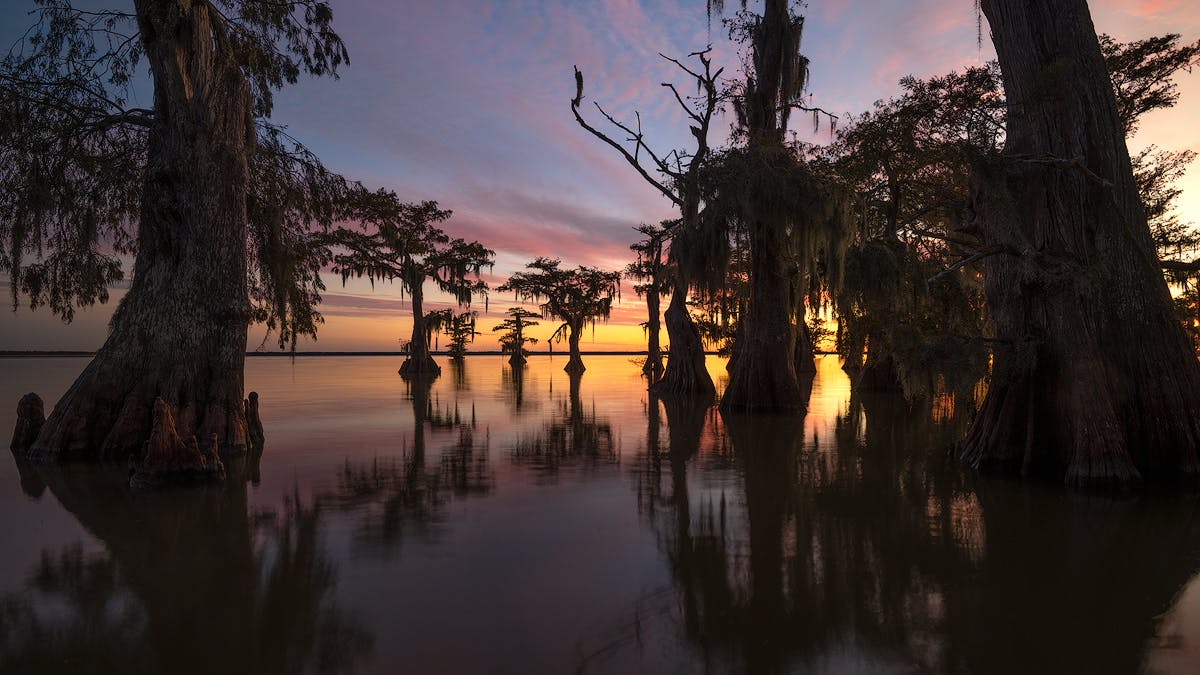The image depicts a serene lakeside or swamp at either sunrise or sunset, with the sky adorned in a soft periwinkle hue intertwined with vibrant pink and gray streaks. At the horizon, the sun emits a rich yellow glow, creating a stunning marbled effect in the sky. The calm water below mirrors the pink and blue tones, producing a tranquil, almost ethereal reflection. Dominating the scene are several hardy-trunked trees with sparse, fuzzy green foliage, their reflections perfectly mirrored in the water's still surface. These trees, some large and leaning as if weighed down, are scattered throughout both the foreground and background, contributing to the image's peaceful, natural beauty. The overall atmosphere is one of quiet elegance, with the interplay of colors and reflections crafting a captivating, picturesque moment in nature.